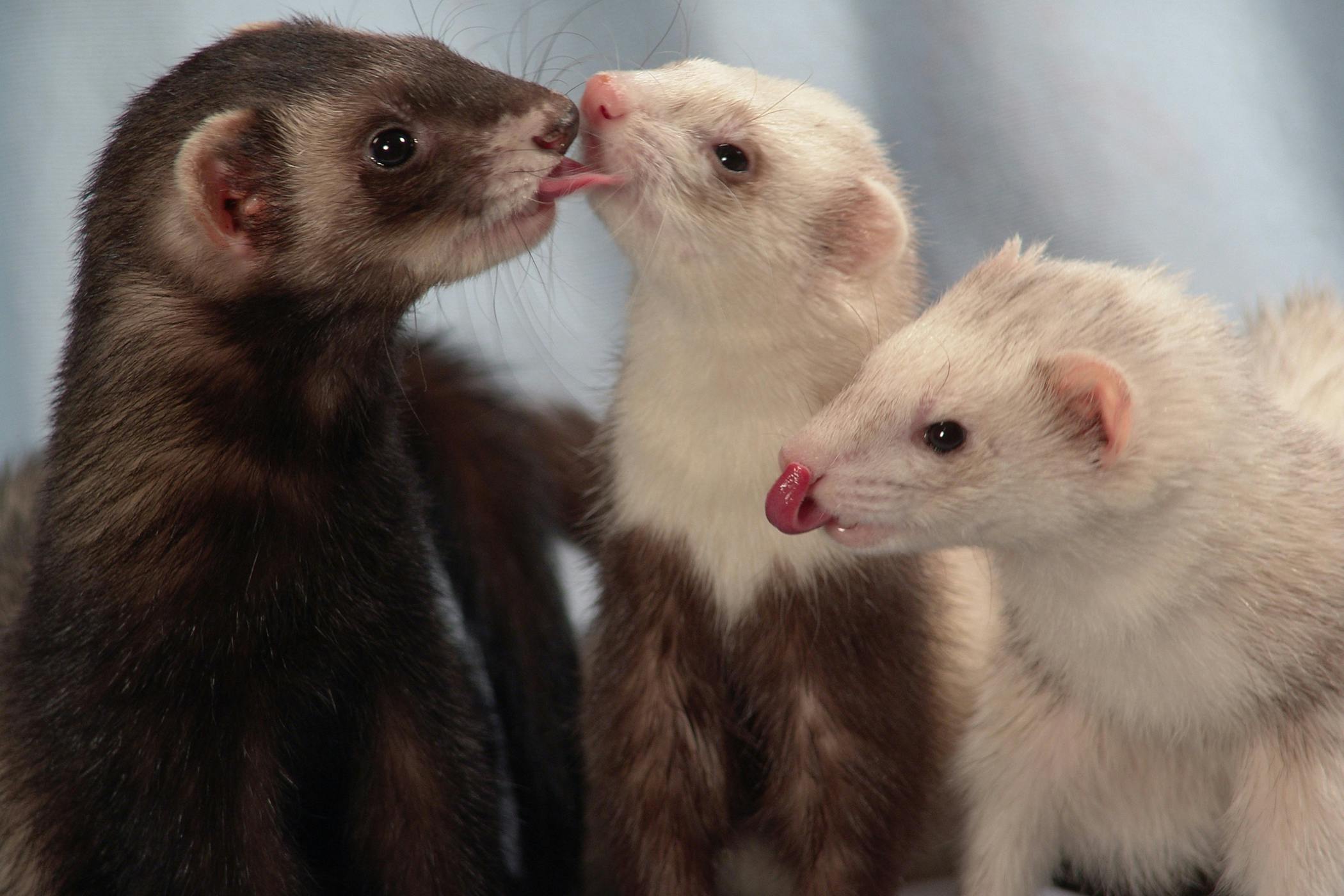In the image, three ferrets with elongated bodies are featured. The ferret on the far left has a dark brown coat and is extending its tongue to lick the face of the ferret in the middle. This middle ferret has a brown body with a white head and neck and is characterized by a pink nose. The ferret on the far right, which is primarily white, also has a white head with a pink nose. All three ferrets have black eyes, giving them a nonchalant appearance as if they are not focusing on anything specific, including the camera. The interaction between the ferrets adds a playful dynamic to the scene, with the leftmost ferret engaging affectionately with the middle ferret, whose head is slightly tilted, while the rightmost ferret’s head is angled downward, gazing away from the group.